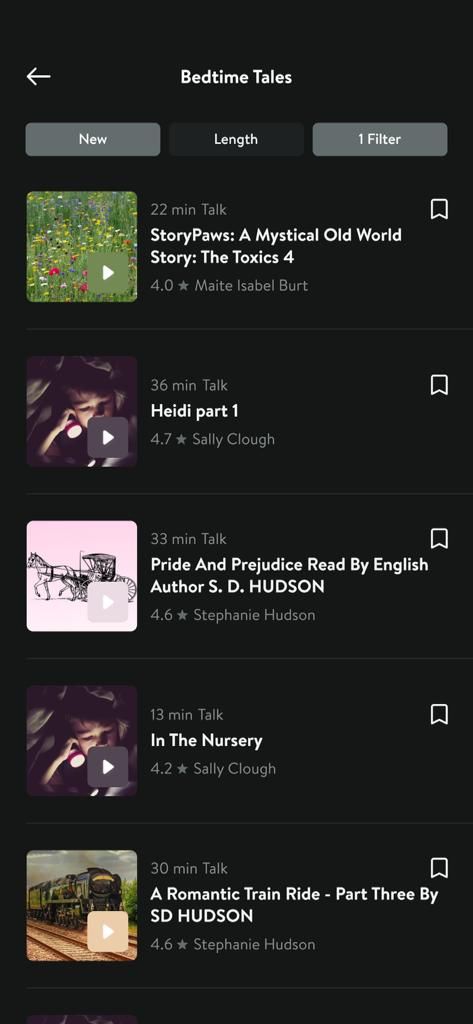The vertical image, captured from a smartphone, features a predominantly black background with no discernible texture or dimension, giving it a flat, one-dimensional appearance. 

In the upper left-hand corner, a white arrow points to the left. Centered in the middle of the image, bold white text reads "Bedtime Tales." Beneath this title are three rectangular tabs. The first tab, shaded in medium gray, displays the word "New" in white letters. The second tab, darker in color and highlighted to show it is selected, reads "Length" in white text. Next to it, in gray, is the note "One Filter."

Below the tabs are thumbnail images representing different audio or video stories, each marked with a play button. The first story, titled "22-Minute Talks," includes a brief description followed by:

- "Story Pause"
- "The Mystical Old World"
- "Story: The Toxics 4"
- Rated Four Stars
- By Mate Isabel Burt

Additionally, there is a small bookmark icon.

The following stories are similarly formatted, with titles, durations, ratings, and authors indicated:

- "Heidi Part 1"
- "Pride and Prejudice," read by English Author S.D. Hudson
- "In the Nursery"
- "A Romantic Train Ride Part 3" by S.D. Hudson